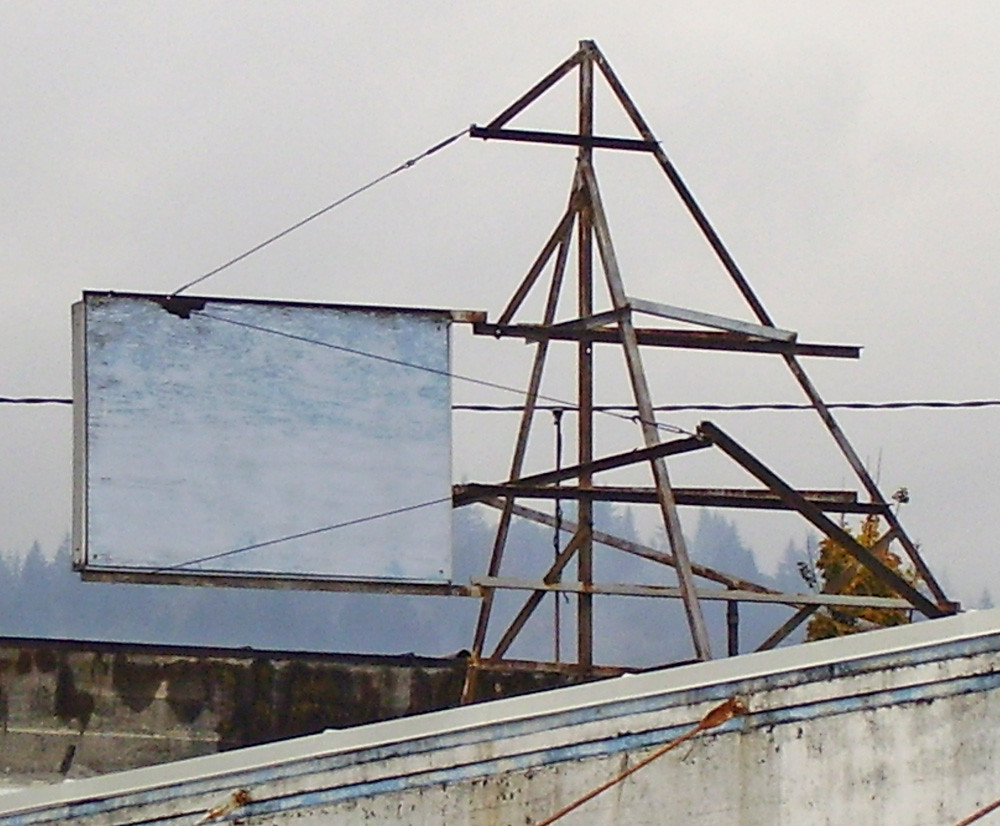The image depicts an outdoor scene featuring a partially constructed billboard or sign, held up by a metal A-frame structure with a triangular design. The frame consists of several thin support beams, including a prominent central beam and angled side beams that give it its characteristic triangular shape. Additionally, smaller beams extend further back along the structure's length. Hanging off the left side is some wiring attached to a piece of plywood. The structure sits atop a building with a tannish-white exterior accented by subtle stripes near the top. At the base of the image is a cement wall displaying a blue stripe and a diagonal red line, further emphasizing the urban rooftop setting. The absence of text on the billboard highlights its incomplete or abandoned state.